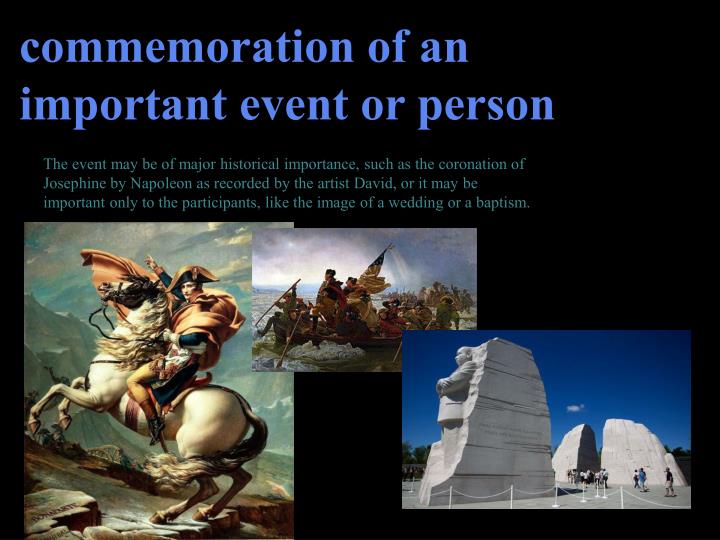The image features a black background with explanatory text at the top in blue script. The main text, split into two lines, reads "Commemoration of an important event or person." Beneath this, in smaller light green text over three lines, it states, "The event may be of major historical importance, such as the coronation of Josephine by Napoleon as recorded by the artist David, or it may be important only to the participants like the image of a wedding or a baptism." Below the text are three distinct images. 

On the left, there is a detailed painting of Napoleon riding a rearing horse, possibly navigating a mountain. The central image appears to depict American settlers or soldiers rowing a boat across a body of water, led by a figure looking ahead determinedly, with their flag visible. In the bottom right, there is a photographic image of monuments, including a prominent statue of a man in a suit crossing his arms, likely Martin Luther King Jr., set against a bright blue sky with tourists milling around.

The overall setting suggests an educational presentation or advertisement, given the structured layout and informative text. The color palette includes shades of white, blue, green, yellow, and brown.